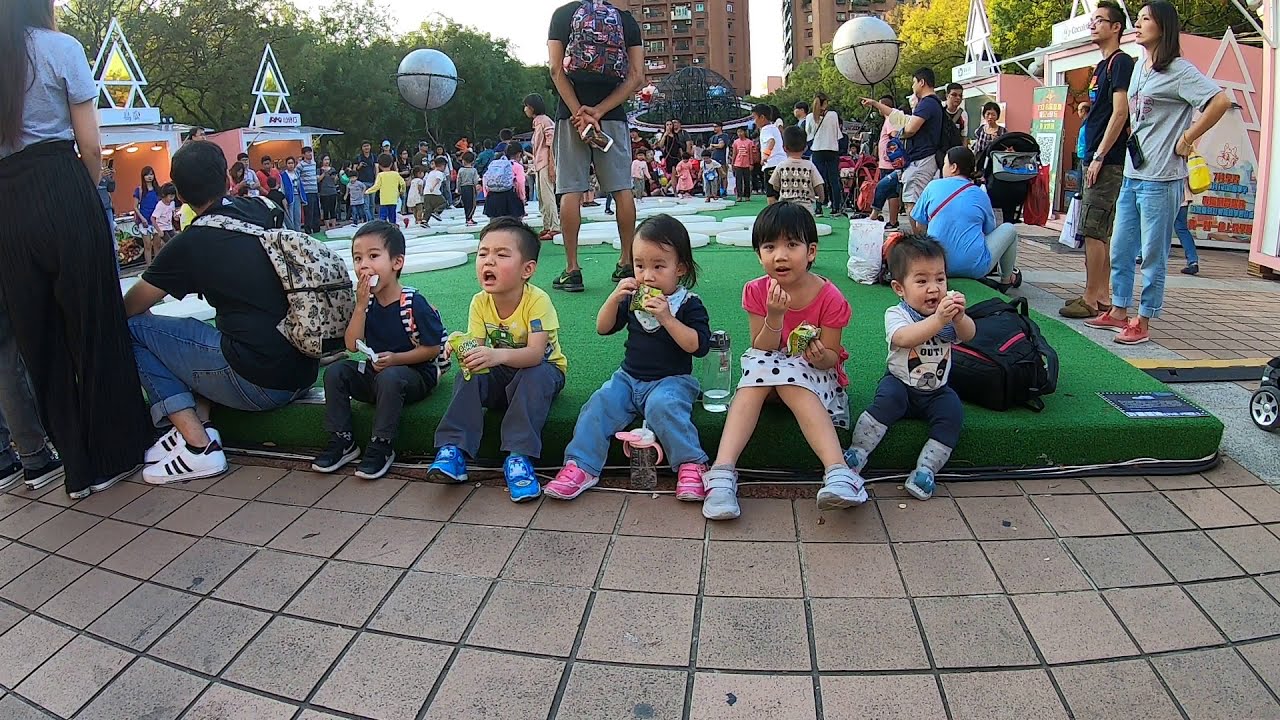In the midst of a bustling urban plaza, a lively celebration or festival unfolds. The scene is dominated by a green, turf-like surface where five children are seated in the center, enjoying snacks. Behind them, throngs of people, including both children and adults, create a vibrant and energetic atmosphere as they run, point, and explore. The background reveals towering high-rises and trees, framing the crowd that gathers around various pop-up venues and tents. Among the attractions are large, planet-themed balloons, including one that resembles Saturn, adding to the festive environment. The bright, sunlit sky bathes the entire setting in a warm glow, while adults watch over the children, ensuring their safety as they play and eat. The vivid hues of pink, white, black, beige, green, light green, yellow, brown, tan, gray, coral pink, and gold enhance the joyous spirit captured in this photograph.